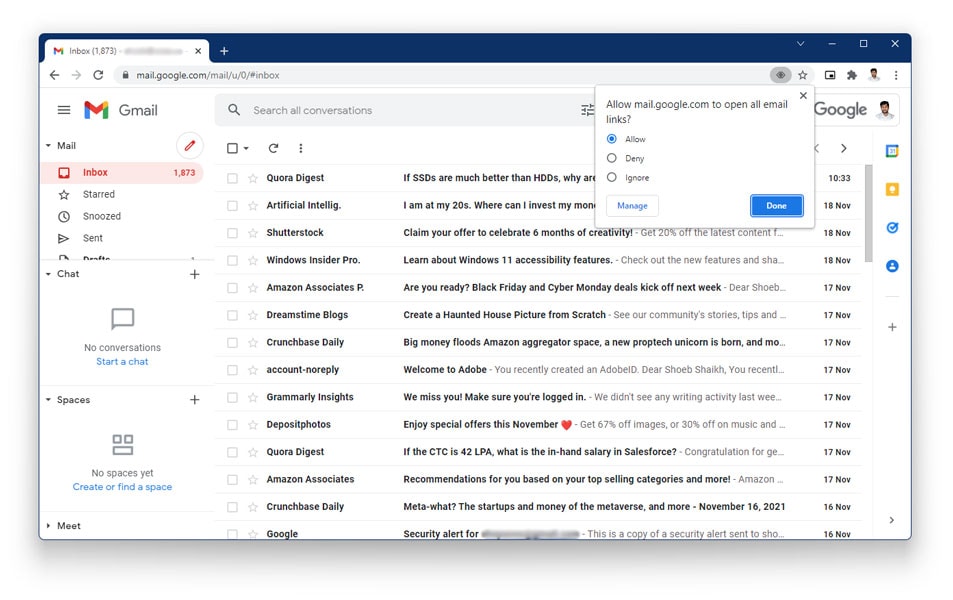A cluttered email inbox is displayed on the screen, showing a total of 1,873 new emails. At the top of the browser tab, the word “Inbox” is prominently visible in black, emphasizing the large number of unread emails. A pop-up message is centered on the upper part of the main screen, asking, "Allow Mail.Google.com to open all email links?" Below this message, three options are listed: "Allow," "Deny," and "Ignore," all written in black text. The option next to "Allow" features a small circle with a blue dot inside, indicating it's selected. Beneath the choices, a blue rectangle with the word "Done" written in white is present, alongside a gray-outlined rectangle containing the blue word "Manage."

The inbox itself has the word “Inbox” highlighted in red, standing out from the rest of the interface. The emails listed include senders such as Quora Digest, Artificial Intelligence, Shutterstock, Windows Insider Pro, and Amazon Associates, with the beginning of each email subject visible in black text. Each email entry has a small rectangle outlined in gray and a gray-outlined star icon next to it, allowing for further management actions. To the far right of the email list, dates like "November 18" are visible, indicating when the emails were received.